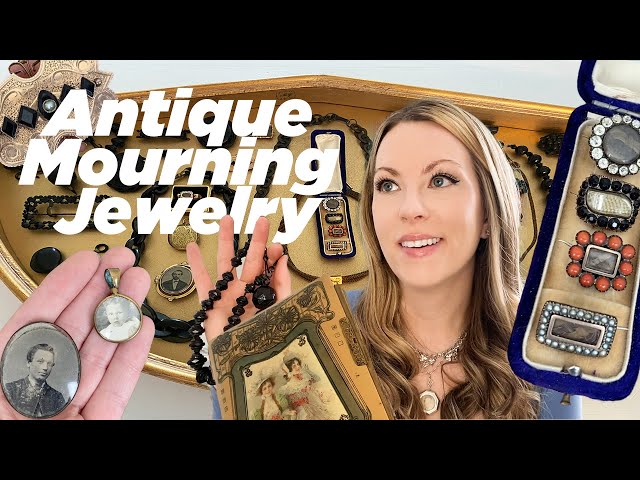The horizontal, full-color image features a detailed layout of antique mourning jewelry, framed by black borders on the top and bottom. In the upper left, white text reads "Antique Mourning Jewelry." The centerpiece of the image is a Caucasian woman with brown hair highlighted with lighter tones, appearing to be in her late 20s to early 30s. She is dressed in a blue top and a necklace, smiling slightly and looking off to the left. The woman holds a golden, book-shaped object that has a portrait of two girls on it along with black beads, resembling a painting or photo pendant.

To her right is a vertically positioned blue jewelry box displaying four pieces of jewelry, likely rings or brooches, each intricately designed with various gems. Positioned in the lower left corner is a hand holding two pendants, featuring black-and-white portraits of a middle-aged man and a young girl. In the background, a brown wooden jewelry box can be seen, filled with various types of jewelry, including necklaces and old photos. The contrasting colors and careful arrangement of items emphasize the theme of antique mourning jewelry, adding a historical and sentimental aura to the image.